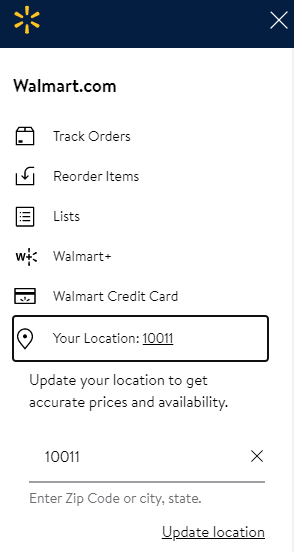Screenshot of Walmart.com Mobile App:

In this screenshot of the Walmart.com mobile app, the top left corner features the distinctive Walmart star icon, with an "X" button also on the left-hand side for easy exit or closure. Below, a well-defined white screen with black text prominently displays "Walmart.com" at the top.

This main screen showcases a comprehensive menu of icons for various functions:
- Track Orders
- Reorder Items
- Shopping Lists
- Walmart Plus
- Walmart Credit Card

Beneath the icons, there is a boxed section displaying your current location, signified by the zip code "10011" which is underlined. The location box is outlined, indicating that it is selected.

A prompt below advises users to "Update your location to get accurate prices and availability." Following this, there is an editable text box pre-filled with the zip code "10011" and an "X" on the right side for quick deletion. 

A gray divider line separates this section from additional instructions: "Enter zip code or city, state." Finally, in the bottom-right corner, an "Update Location" button is available, enabling users to confirm any changes in their location.

This detailed navigation layout ensures users can efficiently manage their shopping preferences and receive accurate local information.